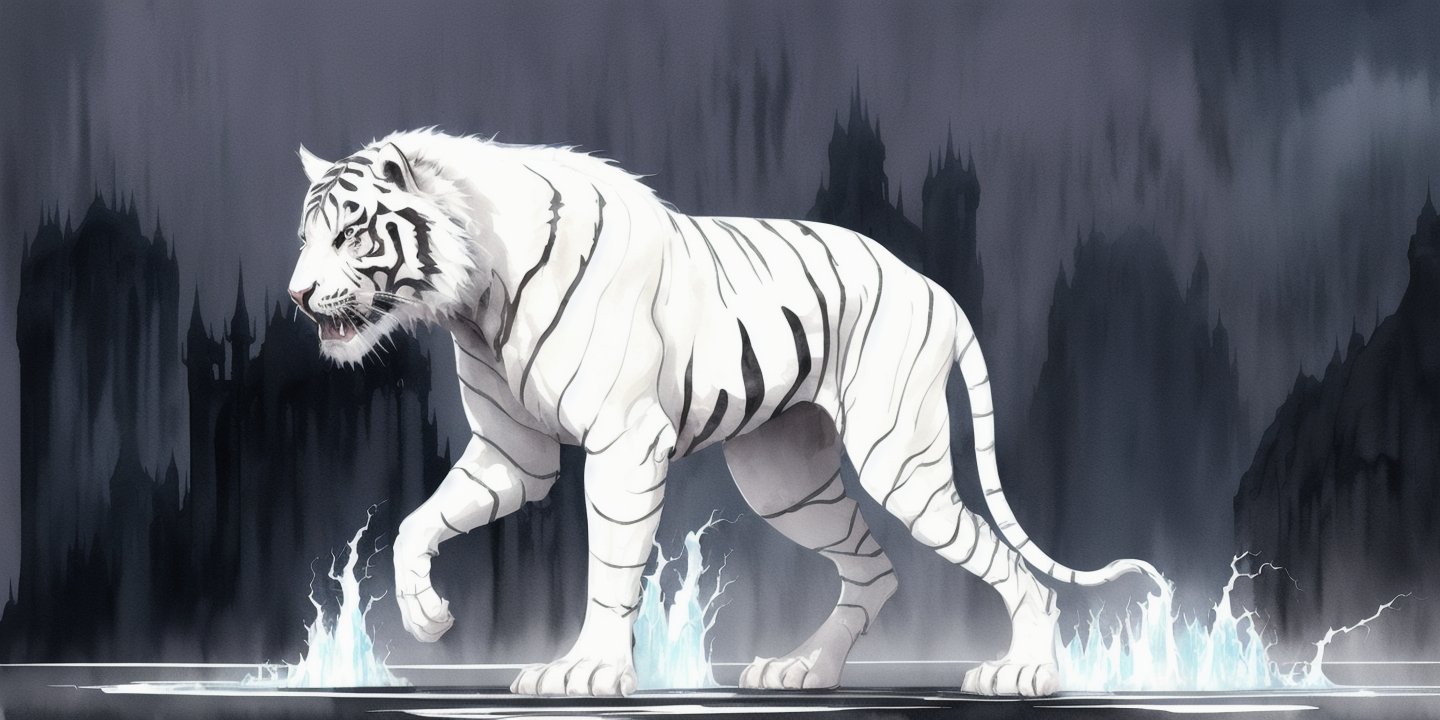The image is a highly realistic and detailed digital drawing of a white tiger with black stripes. The tiger, depicted in mid-walk with its right front paw slightly lifted, exudes a lifelike quality despite being an animated figure. Its mouth is slightly open, showcasing its fangs, adding to its realistic portrayal. Surrounding its paws are dynamic, flame-like streams made of ice, resembling water or electrical currents shooting upwards, which add an intense, almost mystical element to the scene. The tiger is positioned against a background of dark gray and black shades, featuring a smudged, painted effect that evokes a turbulent, almost stormy atmosphere. The tiger appears to be walking on a sleek, glass-like black floor that reflects its majestic form, further enhancing the high-quality and clear presentation of the image.